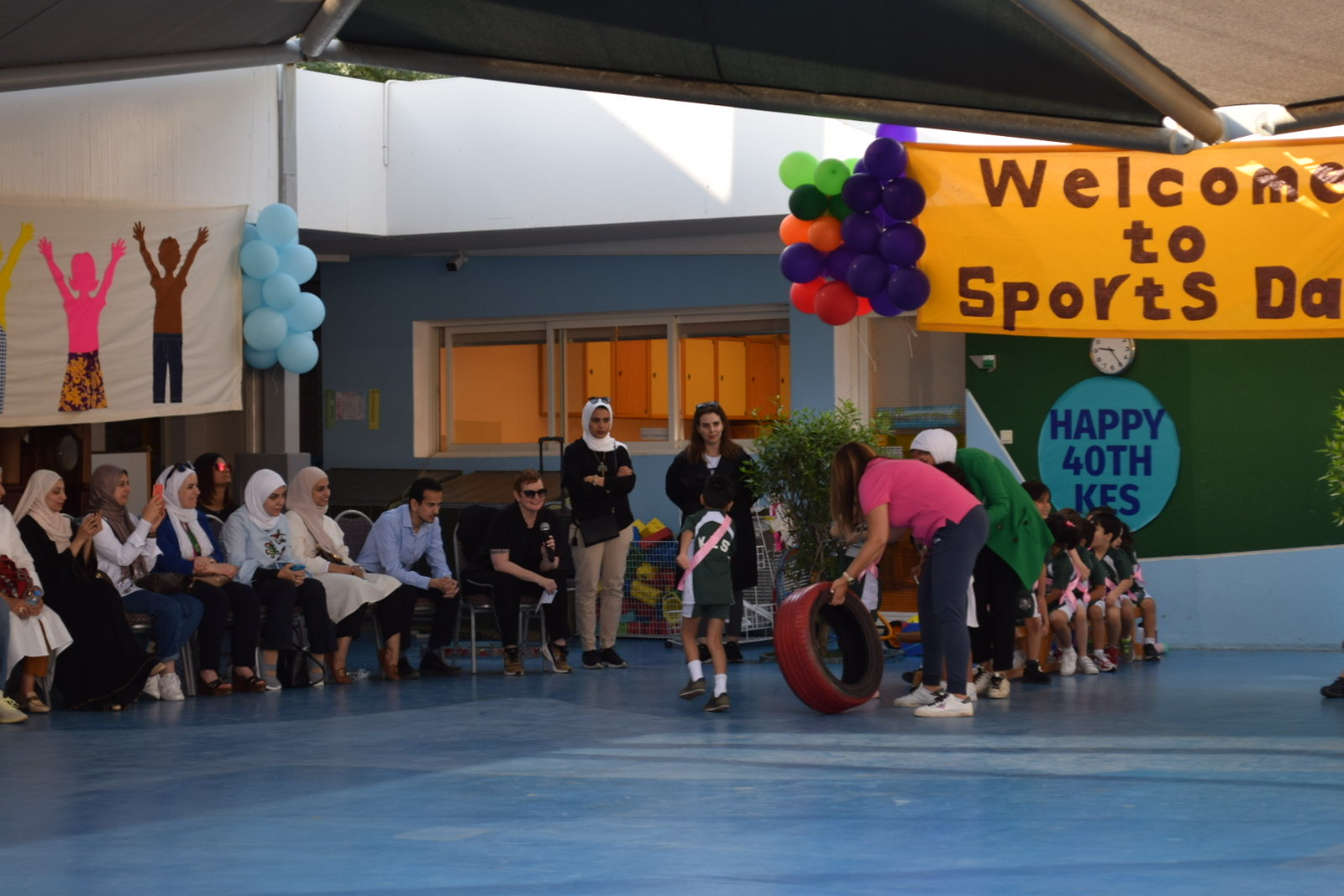A joyous scene unfolds during the 40th anniversary celebration of KES, marked by a vibrant Sports Day event. The image captures the diverse and lively atmosphere, filled with women and children adorned in colorful attire and accessories. Prominently, an orange banner with bold red lettering announces "Happy 40th KES," complemented by a blue circle featuring the same celebratory message in blue text.

Participants, some wearing white and tan head wraps, are seen either seated or standing, engaging in various activities and interactions. A woman in a striking pink shirt stands out, alongside children adorned with pink ribbons. The air is filled with an array of balloons in blue, purple, pink, and green, adding to the festive ambiance. The positioning of individuals varies, with some looking toward others who are walking nearby, though their faces are turned away from the viewer. The setting, likely a school or camp, is abuzz with excitement as everyone comes together to commemorate this milestone event with sports and camaraderie.